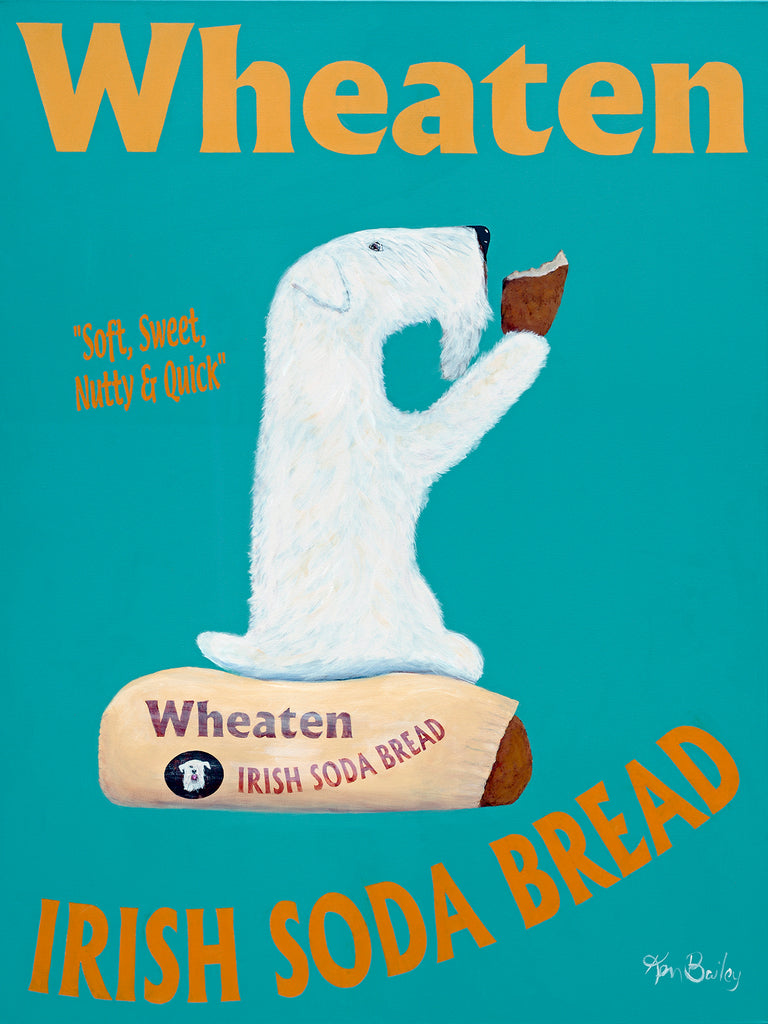This hand-painted advertisement poster for Wheaton Irish Soda Bread features a charming and detailed illustration against a vibrant turquoise background. Central to the image is a small, white terrier-type dog—likely a Schnauzer—holding a partially eaten piece of Irish Soda Bread in its paw. The dog, characterized by its white fur and black nose, is seated on a wrapped loaf of the bread, with the packaging clearly reading "Wheaton Irish Soda Bread" in bold letters. The product name, Wheaton (spelled W-H-E-A-T-E-N), appears prominently in bold orange letters, accompanied by a descriptive quote, "soft, sweet, nutty, and quick." The lower portion of the advertisement features the text "Irish Soda Bread" in a gentle arc. The artwork is neatly signed by the artist, possibly Ken Bailey or a name starting with a G, in the bottom right corner, adding a personal touch to this eye-catching promotional piece.